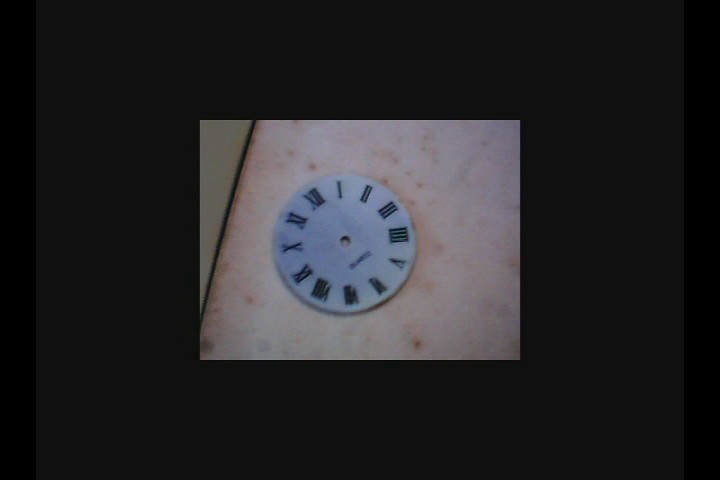In the center of this predominantly black image, a square draws attention with its muted tones. The square features a subtle transition from a beige shade in the upper left corner to a pale pink salmon hue dominating the rest. At its core, a circular element showcases Roman numerals I through XII, reminiscent of a traditional clock face, yet conspicuously devoid of any clock hands.